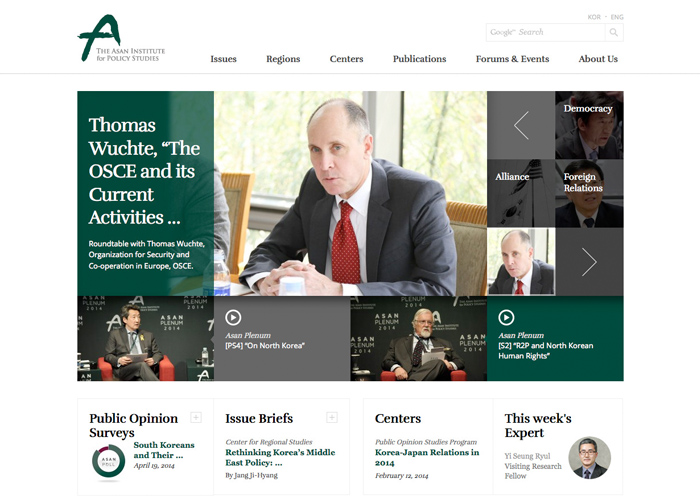**Detailed Caption:**

The image showcases the homepage of the Asian Institute for Policy Studies, resembling a college's informational web portal. The upper left-hand corner features the institute's logo in green on a white background with black lettering. The menu bar includes options for 'Our Issues,' 'Regions,' 'Centers,' 'Publications,' 'Forums and Events,' and 'About Us.' On the upper right-hand side, there is a Google search bar set to English.

Centrally, the page has a distinct section featuring an older balding white man in a business suit with a red tie. His name appears to be 'Thomas Wuchte' associated with OSCE (Organization for Security and Co-operation in Europe) activities. The text mentions a roundtable discussion featuring him.

To his left, there is a mention of 'Democracy' with a left-facing arrow pointing towards the 'Alliance of Foreign Relations.' To his right, another photograph of Thomas Wuchte appears, directing attention with a right-facing arrow toward content on 'Asian Platinum on North Korea' and 'North Korea Human Rights.'

At the bottom of the page, there are sections for 'More Articles,' which include a public opinion survey discussing South Korea’s issues and beliefs, alongside content on Korea’s Middle East policy and detailed views on Korea-Japan relations in 2014. The section also highlights an expert feature for the week: Ying Shing Raul.